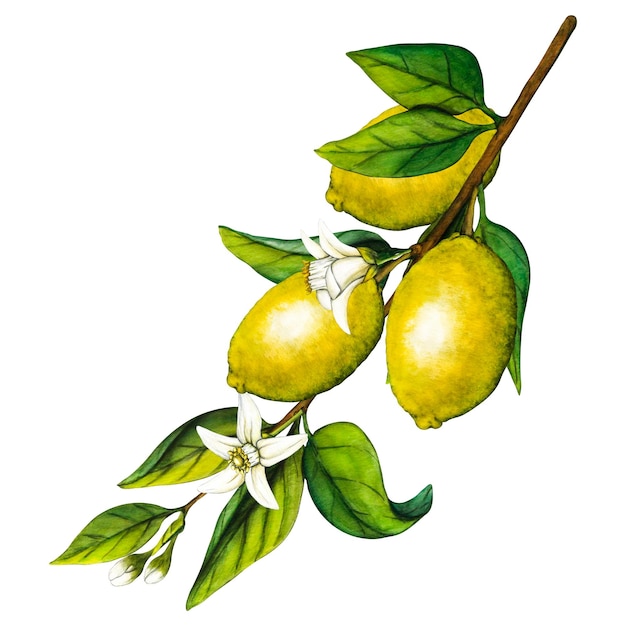The image depicts a detailed, hand-colored drawing of three lifelike, yellow lemons hanging upside down from a brown, curved vine or tree branch. The lemons, which appear dark yet realistic, show light reflections on their rinds. Accompanying the lemons are green leaves positioned at both the bottom and the start of the vine. Interspersed along the vine are small buds and white flowers with yellow stems, some having yet to bloom. The entire scene, against a white background, features meticulous coloration, bringing vibrancy to the lemons, leaves, and flowers.